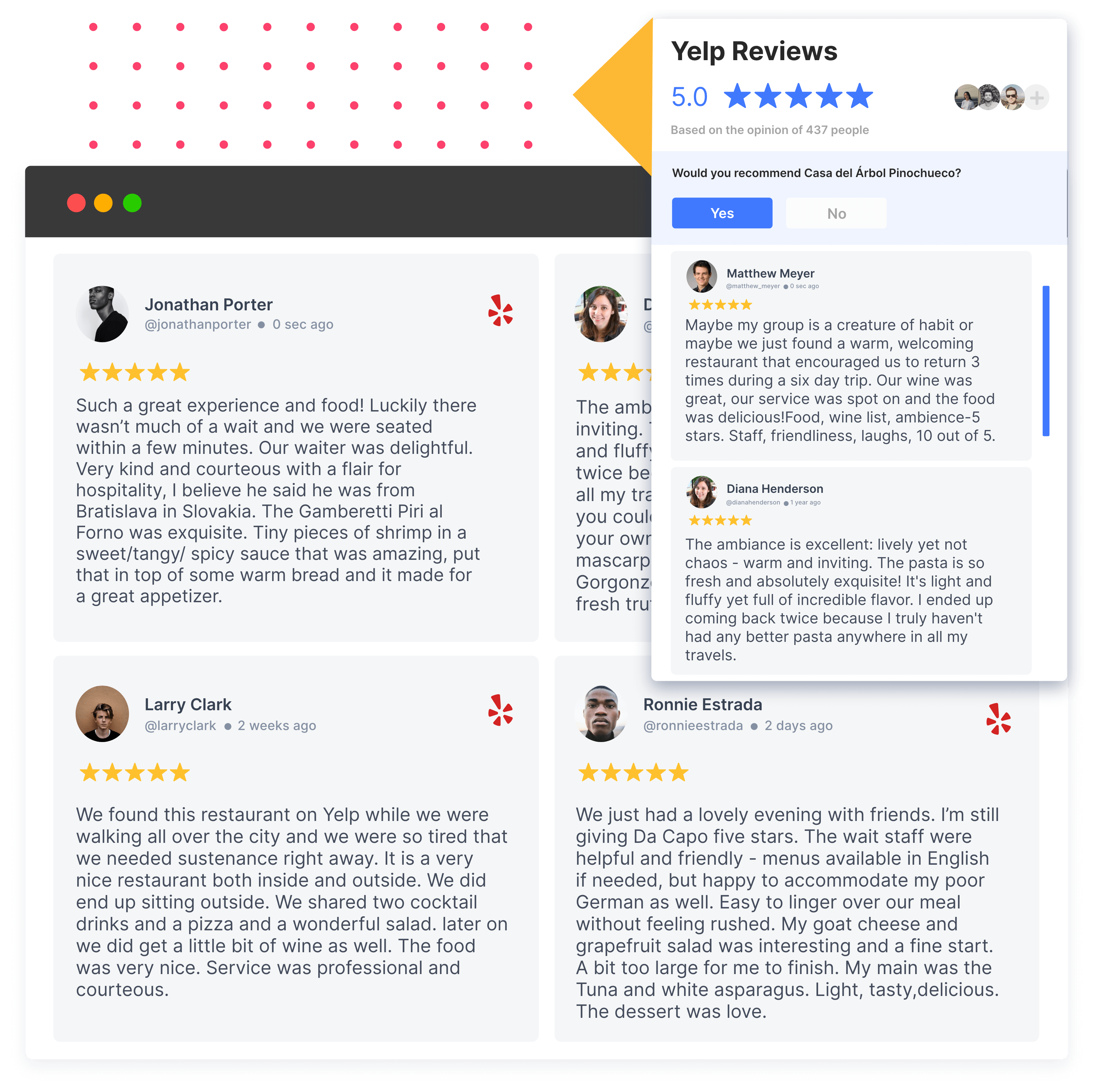The image features four individuals engaged in an intense debate, set against a stark black background. At the top of the image are forty-eight small red dots arranged in a grid-like pattern. In the bottom left corner, there are three larger dots in red, yellow, and green. These larger dots stand out against the dark background. The text on the image reads: "Help Reviews: 0/5 stars," followed by options "View: Yes, No" in bold, black writing. Names mentioned in the caption include Ronnie Nevada, Larry Clark, and Jonathan Perder.